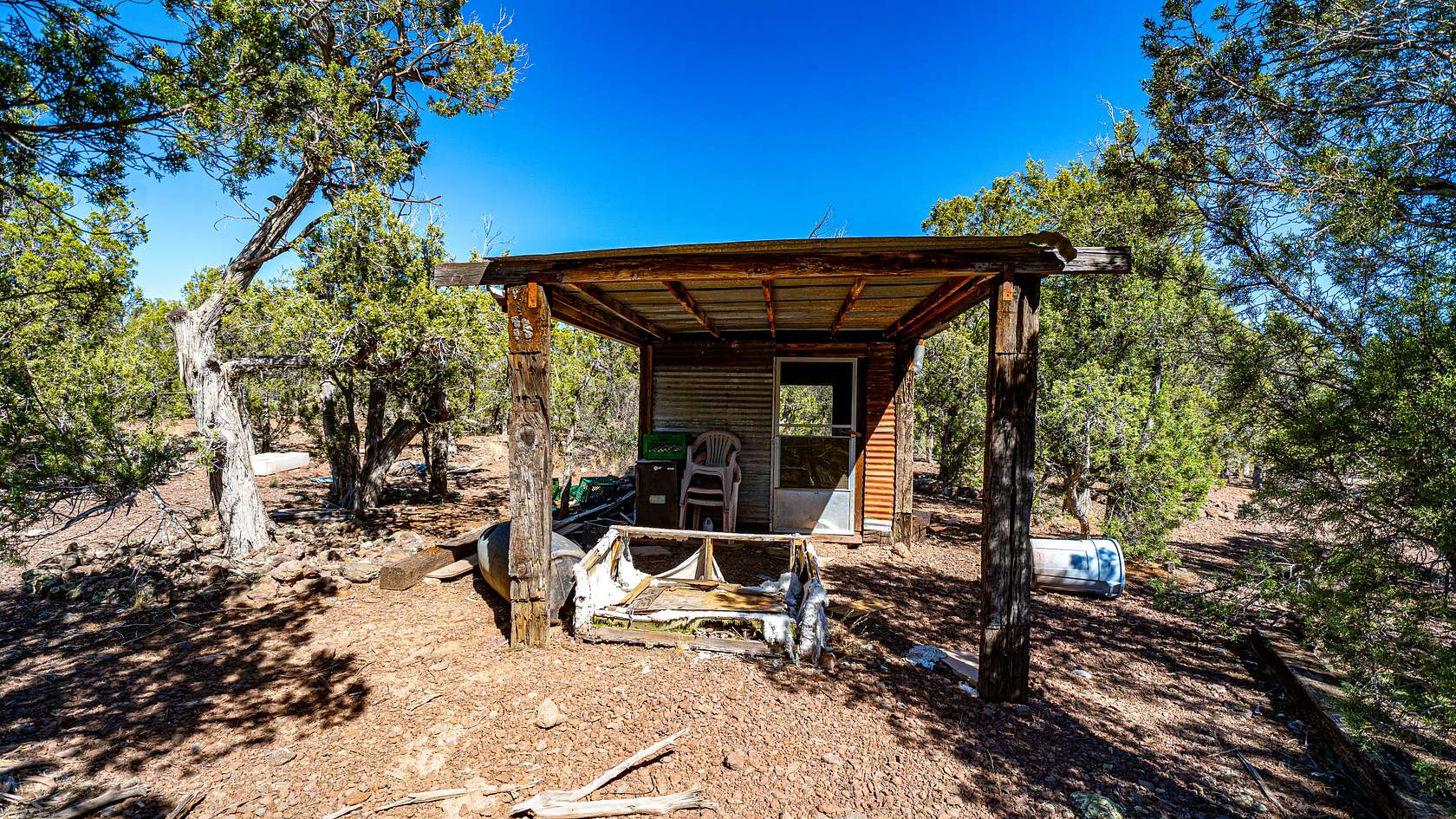This photograph captures a desolate, rudimentary structure, possibly a tiny house, situated in what appears to be an arid woodland or desert landscape, reminiscent of the American Southwest or the Australian Outback. The deep blue sky, which may have a filter accentuating its vivid color, forms a striking backdrop.

The tiny house, positioned at the center of the image, is a simple, run-down wooden cabin with a flat roof. Extending from the front is an awning supported by two sturdy, rough-hewn wooden posts. These posts appear to have carvings, adding a rustic charm to the otherwise decrepit structure. A metal screen door, potentially salvaged, serves as the entrance.

The surrounding area is cluttered and neglected. To the right of the house, a stack of old, inexpensive plastic lawn chairs leans precariously. An overturned trash can and a fallen gray barrel are scattered around the yard, indicating abandonment or neglect. Additionally, there is a broken-down cage or pen in disrepair, suggesting it once housed livestock or chickens.

The ground is a barren, tan, rocky surface interspersed with debris, including what appears to be a cooking device and various other weathered items. Sparse, scraggly trees—both evergreen and deciduous—dot the landscape around the house, adding to the sense of isolation and desolation.

In summary, the image portrays a forgotten, dilapidated tiny home in a stark and dry environment, underscored by a brilliantly clear, blue sky. The scene suggests a life once lived here, now abandoned and overtaken by the elements.